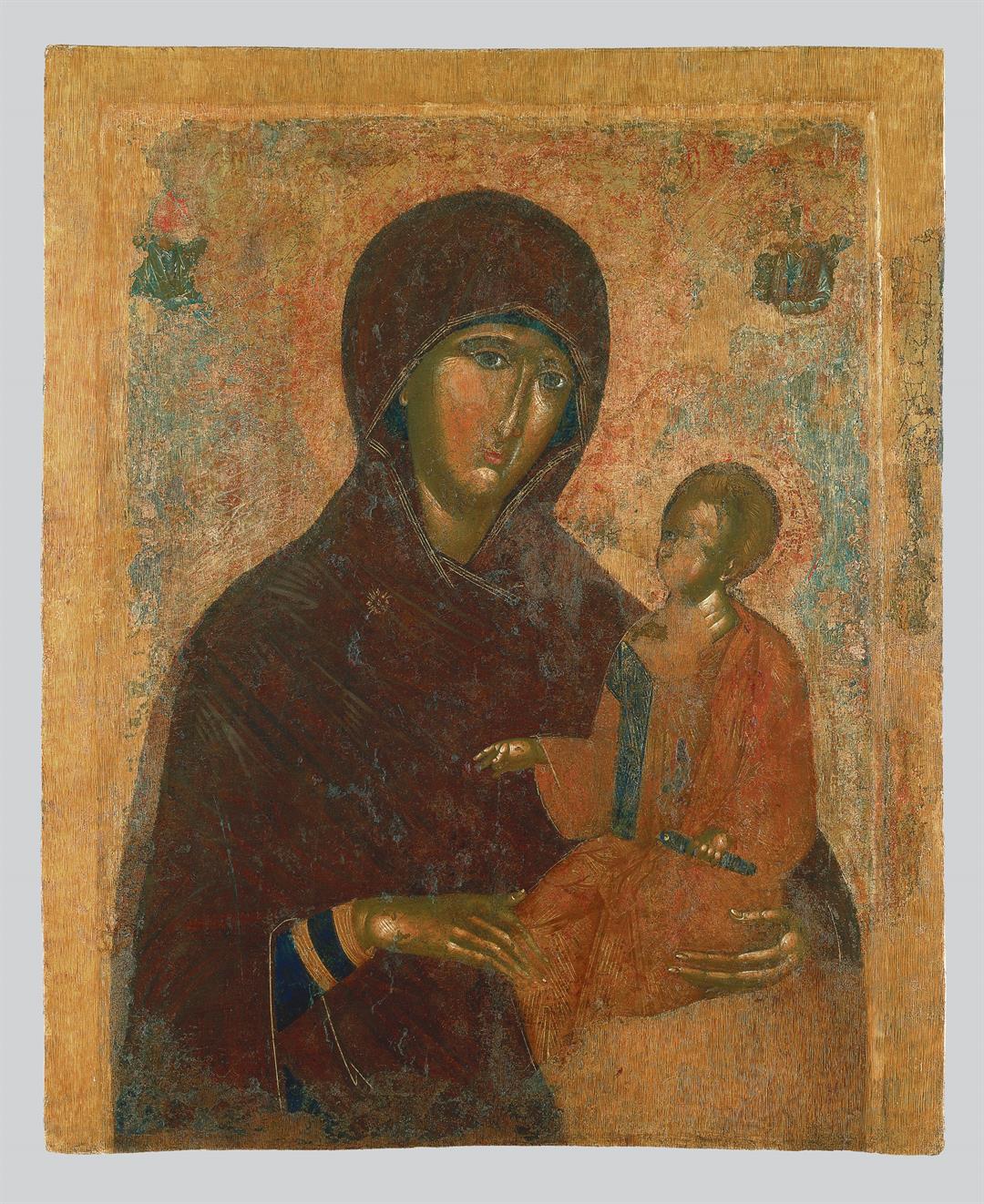This photograph captures an old oil painting, characterized by a gray border that appears to be painted on. The painting predominantly uses a palette of orange, brown, blue, tan, and flesh tones. The background is mainly orange with additional hues of blue and red at the center. Depicted are an adult woman and a child, both facing the viewer. The woman, positioned on the left side, wears a red head cape that flows down to her arms, beneath which a blue and tan or yellow striped sleeve is visible. Her left arm cradles the child, while her right hand rests gently on the child's lap. The child, who sits on the woman's right, is dressed in a long red outfit extending over their feet and wrists, accented with blue. While the woman's face is clearly visible, the child's face remains blurry. The individuals are dressed in what appears to be fancy or elaborate clothing, suggesting a setting or period worthy of a museum display. No text is present in the image.